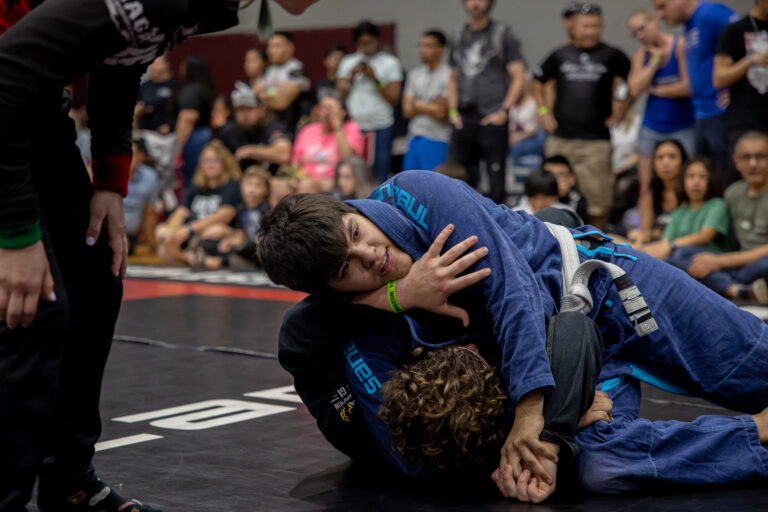This photograph captures an intense moment in a high school wrestling match on a black mat. Two teenage wrestlers, both in blue uniforms but slightly different shades, grapple with each other. The wrestler on top, who appears younger, is in a dominant position, securing his opponent's arm behind his ear. He is distinguished by a white belt tied around his waist. The competitor beneath him is nearly on his back, straining against the control. On the left side of the image, a referee, who seems to be a woman with white-painted nails, is closely examining the match to determine if a pinfall is imminent. She is dressed in a black outfit with red and green wristbands. In the background, a blurry mix of spectators—children, teenagers, and adults, some sitting on the floor and others standing—watch the match with rapt attention. The palpable tension of the match is contrasted by the slight smile on the dominant wrestler's face, hinting at his confidence in victory.